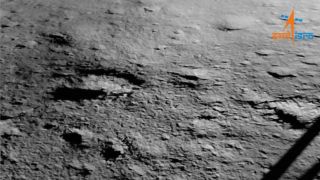This is a very small, low-resolution black-and-white image of the moon's surface, likely a snapshot or screenshot. The image features a variety of crater textures, with some larger and some smaller, on a rocky, bumpy terrain that includes small rocks, loose gravel, and dirt, lending it a vintage appearance. In the upper right corner is an indistinct logo that is half orange and half blue, though its text is unreadable due to the image size. In the bottom right corner, there are two shadowy bars or shapes adding an intriguing mystery to this already enigmatic and diminutive picture. Given its tiny size, it seems more suitable as a profile picture or thumbnail but fails to clearly convey detailed information about its subject.